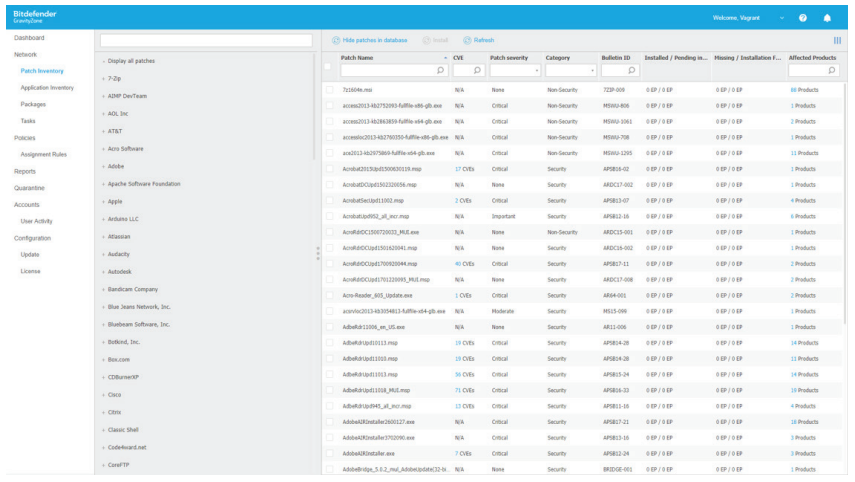The image features a densely-packed user interface of an application with several distinct sections. In the top right corner, there is a blue header, though the text within it is obscured and unreadable. Below this header, the upper left corner displays another block of text that is similarly indiscernible due to its small and blurry nature. Directly beneath this text is a menu presented against a white background, containing approximately 15 selectable options, one of which is highlighted in blue.

To the right of this menu, there is a text box, and directly below it, a list of items arrayed against a light gray background. Each item is presented with a number on the left and an associated name on the right. Adjacent to these items are two search bars positioned at the top, followed by two drop-down menus. Further down, there is another search bar flanked by two empty spaces and an additional search bar at the bottom.

The lower portion of the image showcases another list of items, organized into eight columns, all filled with text that cannot be deciphered due to the image’s quality. The overall layout appears to be data-intensive, likely intended for detailed information management or navigation.